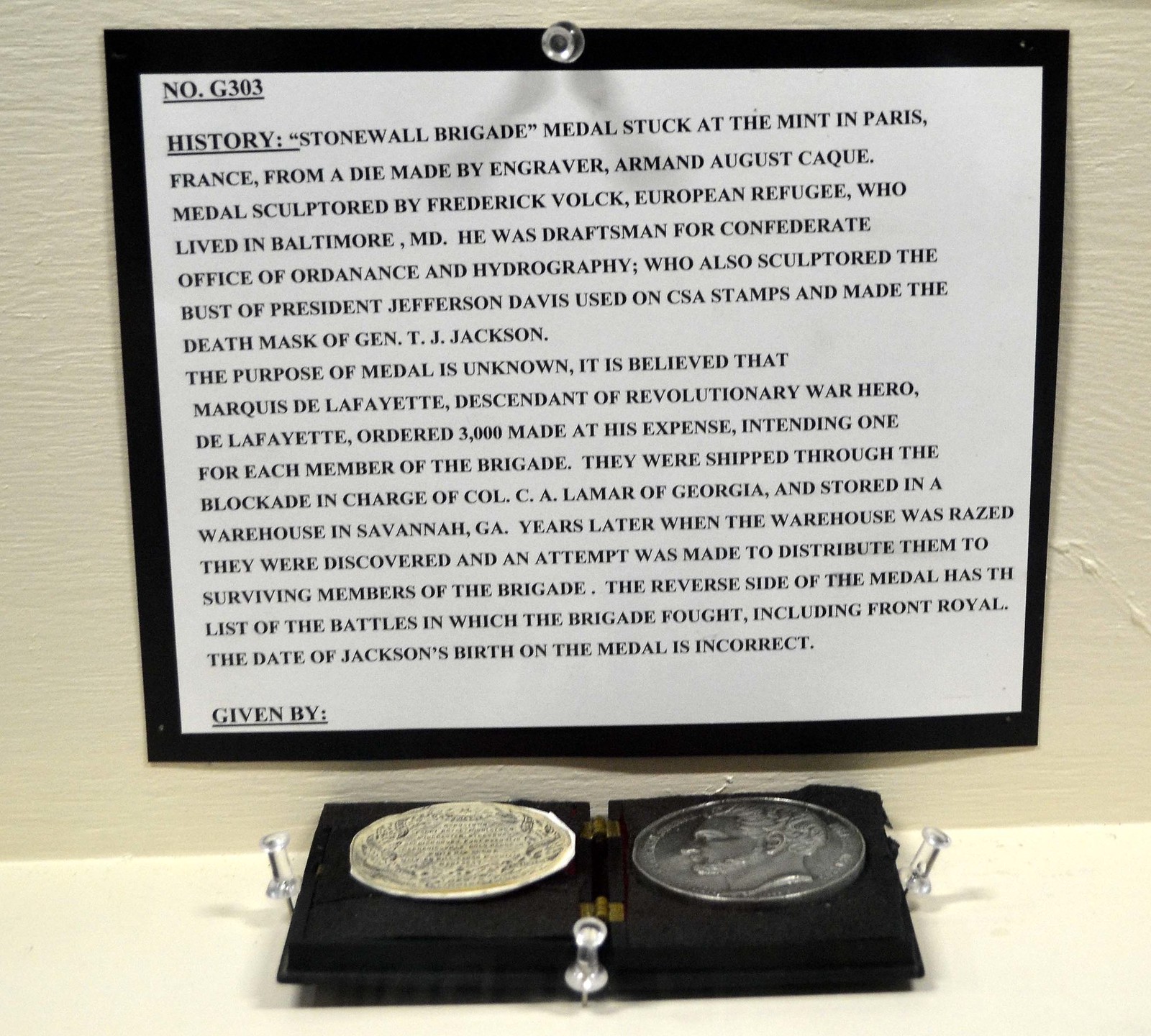This is a horizontally oriented rectangular photograph displaying a printed historical story written entirely in all caps, in Times New Roman font, black on white. The text is tacked to a white wall that features a crisscross pattern. The document has a black border and measures approximately 5 by 10 inches. To its left, there's an underlined label reading "No. G393". Following a line space, the left-aligned text underlines the word "HISTORY" and discusses the "Stonewall Brigade".

Beneath the document, resting on a horizontal white surface, is a black rectangular display case showcasing two large coins. One coin resembles a nickel, while the other appears more ornate, possibly of foreign origin. The display case is flanked by clear tacks with metal push parts, and one more tack is positioned at the front, which is either clear or silver. These tacks have dual-tier grips on their tops.

The printed passage elaborates that the coin was struck at the Paris Mint from a die by the engraver Armand Auguste Caqué, and sculptured by Frederick Volk, a European refugee and drafter for the Confederate Office of Ordnance and Hydrography. Volk also sculpted a bust of President Jefferson Davis, which was used on CSA stamps, and created the death mask of Gen. T.J. Jackson. The text indicates that the purpose of the medal remains unknown but speculates it was ordered by Marquis de Lafayette for the Stonewall Brigade. The medals were shipped through a blockade and stored in a Savannah, Georgia warehouse. When the warehouse was demolished, the medals were discovered and efforts were made to distribute them to the brigade’s surviving members. The reverse of the medal lists battles fought by the brigade, although Jackson's birth date on the medal is incorrect. At the bottom left, the document notes, “GIVEN BY:” followed by underlined space.

This item appears to be part of a museum display focused on Civil War-era history, particularly the contributions and memorabilia associated with the Confederate side.